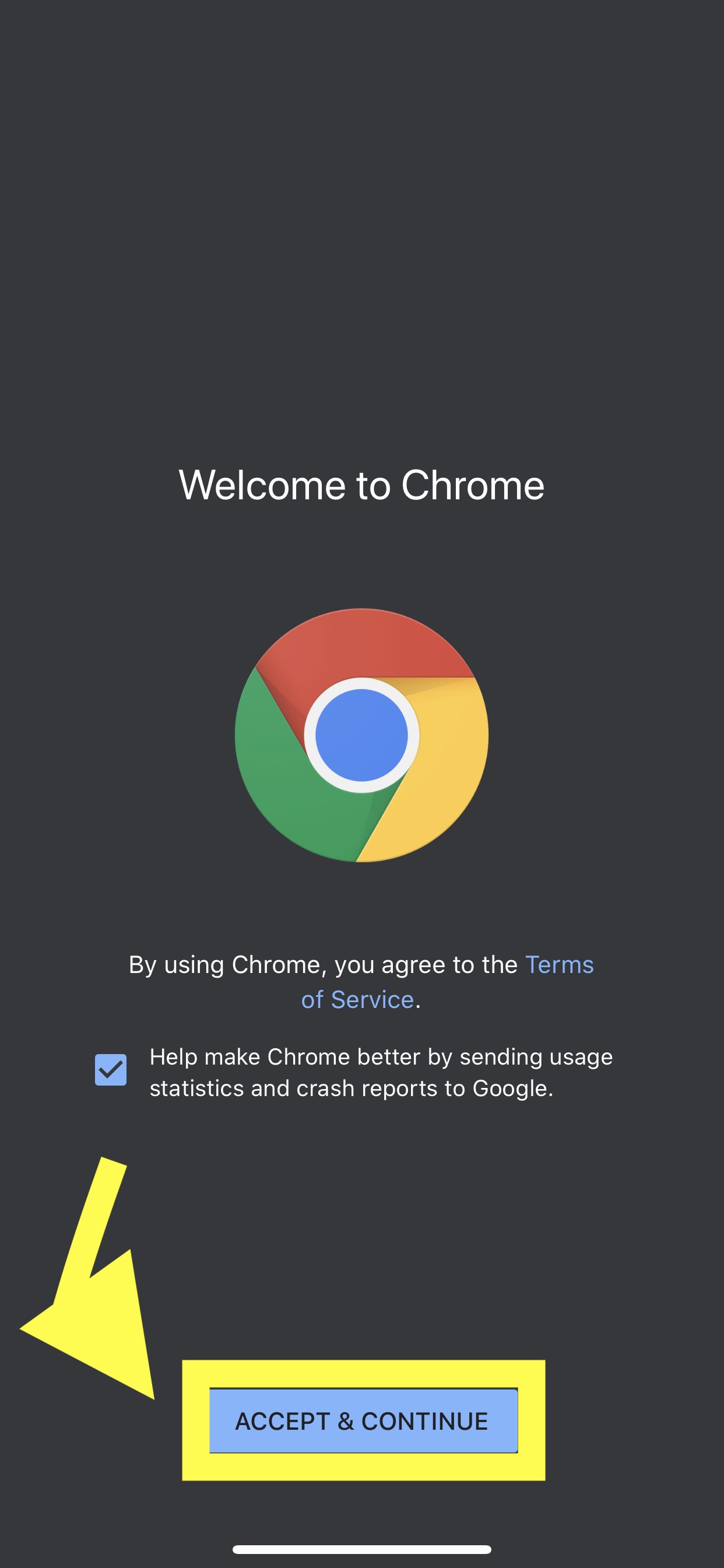The image features a long, sleek black box with detailed text and graphical elements. At the top of the box, approximately four inches from the edge, the phrase "Welcome to Chrome" is prominently displayed in white text. Below this greeting, the iconic Google Chrome logo is centered. This logo consists of a vibrant red section at the top, with green to the left, yellow to the right, and a central blue circle outlined in white.

Underneath the logo, there is a clear statement: "By using Chrome you agree to the Terms of Service," with "Terms of Service" highlighted in blue, indicating it's a clickable link. Beneath this agreement statement, a small blue checkbox is marked with a check. Next to this checkbox, the text reads: "Help make Chrome better by sending usage statistics and crash reports to Google."

To the left side of the box, a large yellow arrow, resembling an upside-down triangle, points downward and slightly to the right. This arrow serves to draw attention to a smaller blue rectangle within a yellow-outlined rectangle, containing the phrase "ACCEPT AND CONTINUE" in bold, capitalized black text.

Approximately two inches below all these elements, a small horizontal white line spans the width of the box, providing a subtle visual break. This composition guides the user through the terms of service acceptance process with clear, visually-distinct elements.